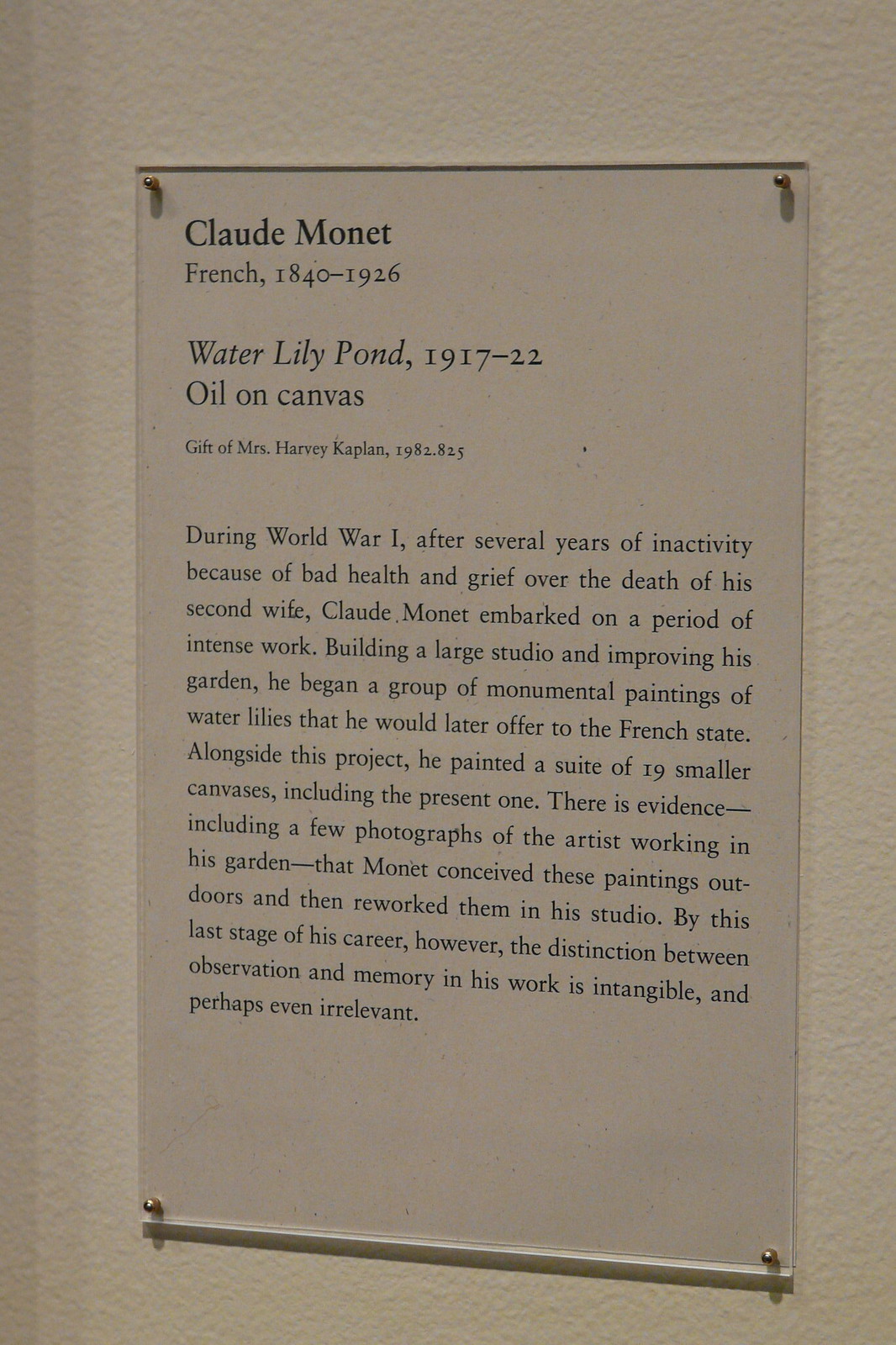The image shows a see-through plaque mounted on a white pebbled wall with four rounded metal screws at each corner. The plaque features black print that reads:

**Claude Monet**  
*French, 1840-1926*  

*Water Lily Pond, 1917-22*  
*Oil on Canvas*  

*Gift of Mrs. Harvey Kaplan, 1982.825*  

Below this information, there is a descriptive paragraph:

"During World War I, after several years of inactivity because of bad health and grief over the death of his second wife, Claude Monet embarked on a period of intense work. Building a large studio and improving his garden, he began a group of monumental paintings of water lilies that he would later offer to the French state. Alongside this project, he painted a suite of 19 smaller canvases, including the present one. There is evidence, including a few photographs of the artist working in his garden, that Monet conceived these paintings outdoors and then reworked them in his studio. By this last stage of his career, however, the distinction between observation and memory in his work is intangible and perhaps even irrelevant."